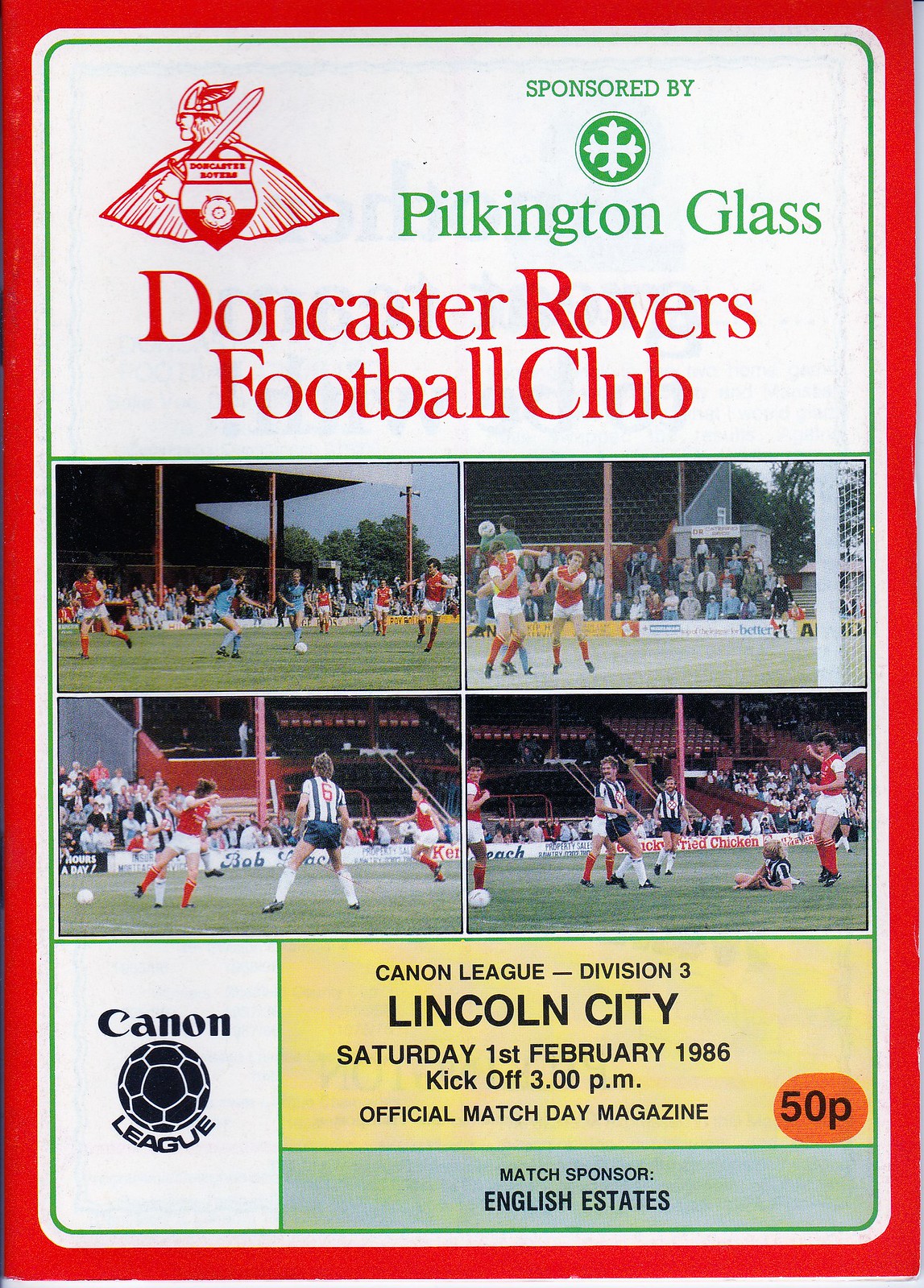Here's a cleaned-up and detailed caption for the given image:

"A vintage soccer program cover prominently features a red background with white text, centering around the Doncaster Rovers logo. The emblem depicts a figure in a cape with a helmet and long hair, looking leftward, and holding a shield and a sword. 'Doncaster Rovers' is written above in green text. The program is sponsored by Pilkington Glass, whose circular logo appears in the center. The text 'Doncaster Rovers Football Club' is displayed in red below.

In the middle, there are four action-packed pictures of soccer players. The bottom left corner highlights the 'Canon League' logo, showing a soccer ball and the Canon camera company brand. To the right, a yellow box indicates match details: 'Canon League Division 3, Lincoln City, Saturday 1st February 1986, Kickoff 3 p.m., Official Match Day Magazine.' The magazine price, '50p,' is mentioned in the bottom right corner of the yellow box. Another green box at the bottom right names 'English Estates' as the match sponsor."